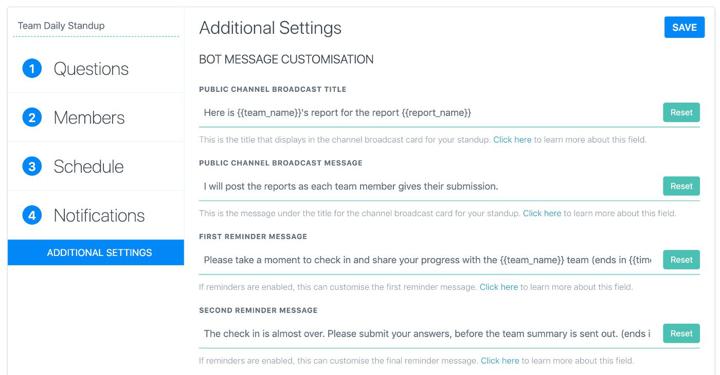This image is a screenshot of an unknown website, featuring various text elements and interface options. On the left side is a vertical menu listing: "Team Daily Standup," followed by sub-options titled "Questions," "Members," "Schedule," and "Notifications." Adjacent to the menu is a blue rectangle labeled "Additional Settings."

Within "Additional Settings," there are sections for "Bot Message Customization" and "Public Channel Broadcast Title." Below these headings, the text specifies: "Here is the team names report for the report." Under "Report Name," it clarifies that this will be the title displayed in the channel broadcast card for standups, accompanied by a hyperlink titled "Click here to learn more about this field."

Further down, under the "Public Channel Broadcast Message," it states: "I will post reports as each team member gives their submission," explaining that this message appears under the title on the broadcast card for the standup, again with an option to learn more.

The section labeled "First Reminder Message" contains the text: "Please take a moment to check in and share your progress with the [team name] team." This message is customizable if reminders are enabled, with another link provided for more information.

Under the "Second Reminder Message" heading, it reads: "The check-in is almost over. Please submit your answers before the team summary is sent out," highlighting that this too can be customized when reminders are enabled, with a link for additional details.

The image is entirely text-based without any illustrative or photographic content, and no people are depicted.